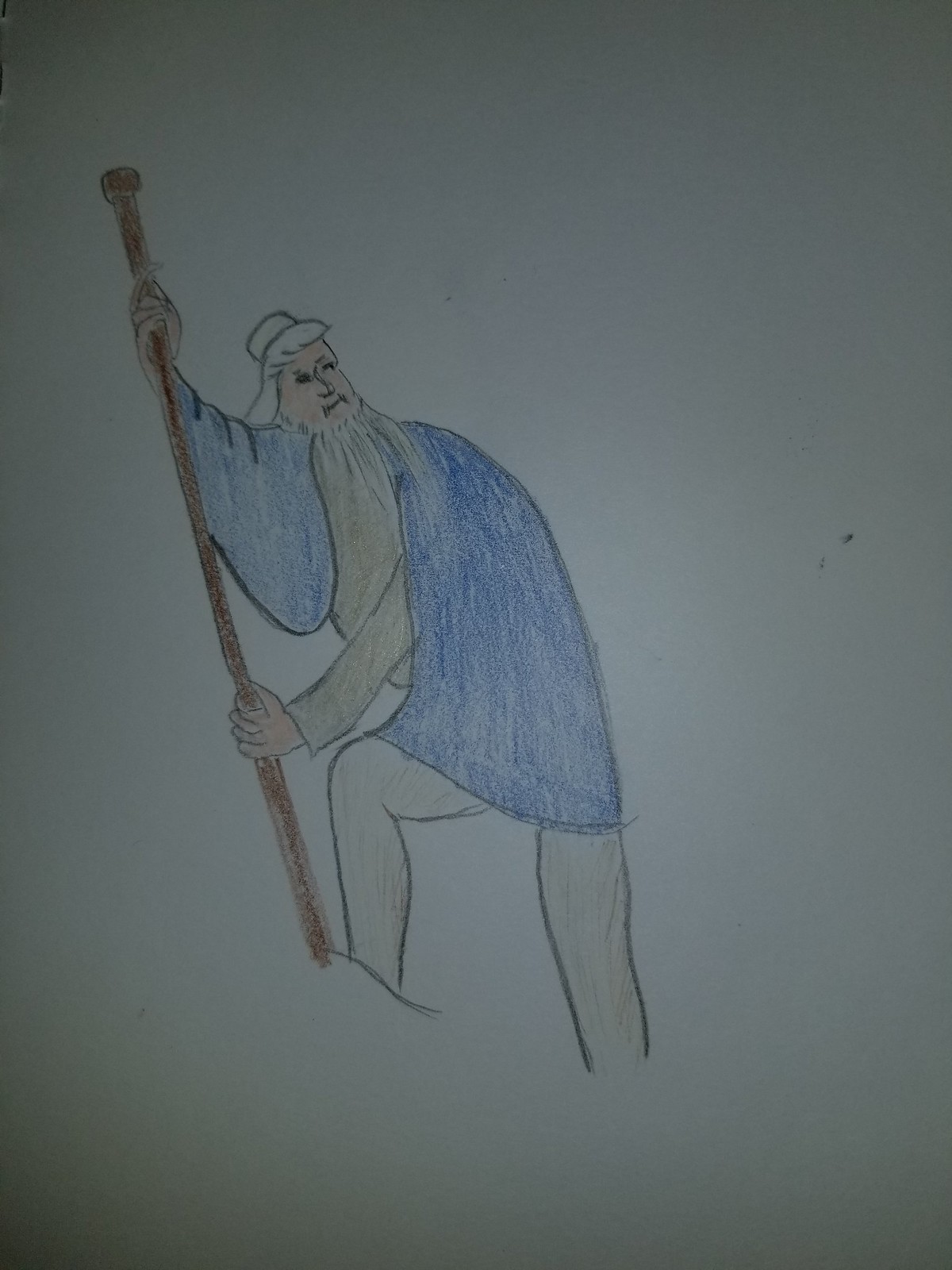This image features a detailed drawing of a man positioned at the center against a plain white background. The man, who appears to have white hair and a long beard cascading down to his chest, is gazing towards the upper right corner of the frame. He is grasping a brown staff with both hands; his right hand firmly holds the upper part of the staff, while his left hand secures the lower part. The man is adorned in a blue top, which adds a touch of color to the otherwise monochrome setting. His legs are visible, complementing his overall attire and stance.